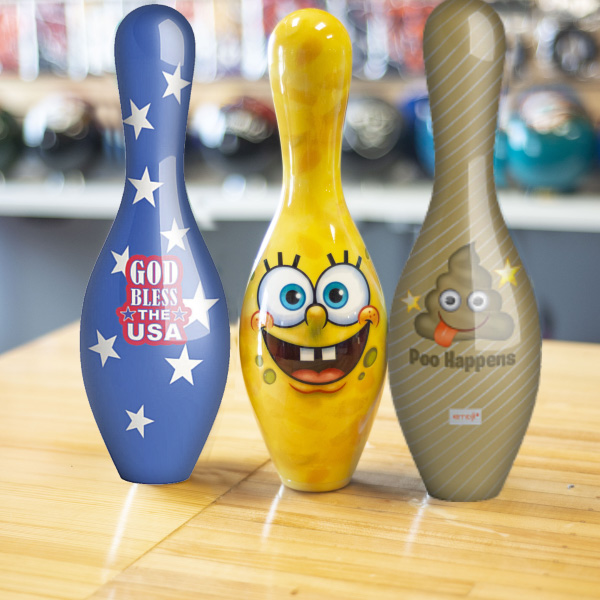In this image, there are three distinctive bowling pins, each showcasing unique and vivid designs, placed on a bright brown wooden table. The background is blurred, but hints of teal, blue, gray, red, and dark green bowling balls suggest it could be a bowling alley.

On the left is a sky-blue bowling pin adorned with white stars and a central white text outlined in red that reads "God Bless the USA," accompanied by two blue stars. The middle pin is yellow, featuring the face of Spongebob Squarepants, complete with blue eyes, eyelashes, an open smiling mouth, and two prominent front teeth. The rightmost pin is brown with thin gray vertical stripes, displaying a poop emoji with big circular eyes, a smiling face, and a red tongue sticking out, captioned with the phrase "Pooh Happens" in black text. Below this, there's an illegible gray square. This quirky set of bowling pins is set against what appears to be a typical bowling alley, given the assortment of colorful bowling balls visible in the distance.